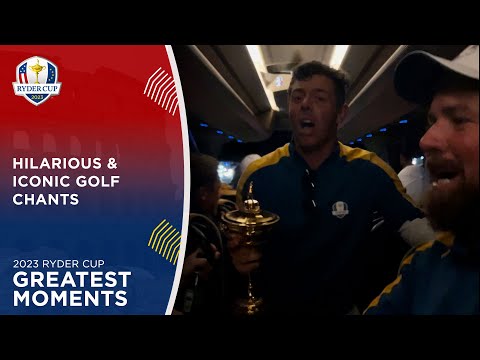The image displays a screenshot from a television broadcast, likely from a sports network, depicting a segment titled "Hilarious and Iconic Golf Chants - 2023 Ryder Cup Greatest Moments." The left portion of the image features an infographic with a red-to-blue gradient backdrop, prominently displaying the event title "2023 Ryder Cup" and its description in white text.

On the right-hand side, the scene includes a slightly dark photograph of two men, both dressed in polo shirts. One man is wearing a hat, while the other, bare-headed, is holding a gold trophy. This trophy has a thin shaft with a flared base and a spherical top encircled by rings, resembling the Earth with its rings. Both men appear to be engaged in chanting or singing, potentially during a celebratory moment. The image composition is letterboxed, with black bars occupying the top and bottom 10-15% of the frame.